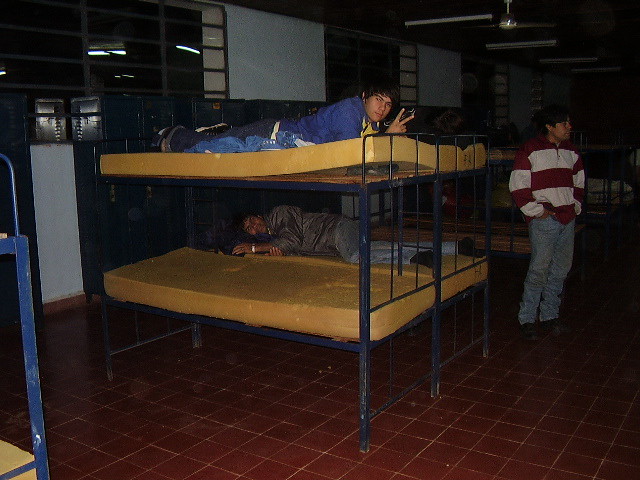A photograph captures the interior of a dimly lit dormitory-type room with a stark, industrial atmosphere. The floor is covered in reddish-brown tiles with visible white grout, and the walls are lined with old, metallic lockers. The room is filled with blue metal bunk beds, each topped with bare, thick yellow foam mattresses devoid of any bedding.

At the center of the image, two blue bunk beds are pushed together. On the top bunk, a teenage boy with short, dark hair lies on his stomach, wearing jeans and a blue sweater. He looks directly at the camera, flashing a peace sign with his fingers. Below him, on the bottom bunk, another boy is lying down, dressed in a grey jacket, blue jeans, and black socks; a watch is visible on his left wrist. At the foot of the bunk bed, a third boy stands in blue jeans and a red and white striped long-sleeved shirt, gazing off to the side. 

The overall ambience of the room is somber and sterile, resembling a hostel, boarding school, or possibly a detainment facility, though the exact nature of the location is unclear. There is a certain forlornness to the scene, emphasized by the neglected appearance of the mattresses and the lack of personal belongings.